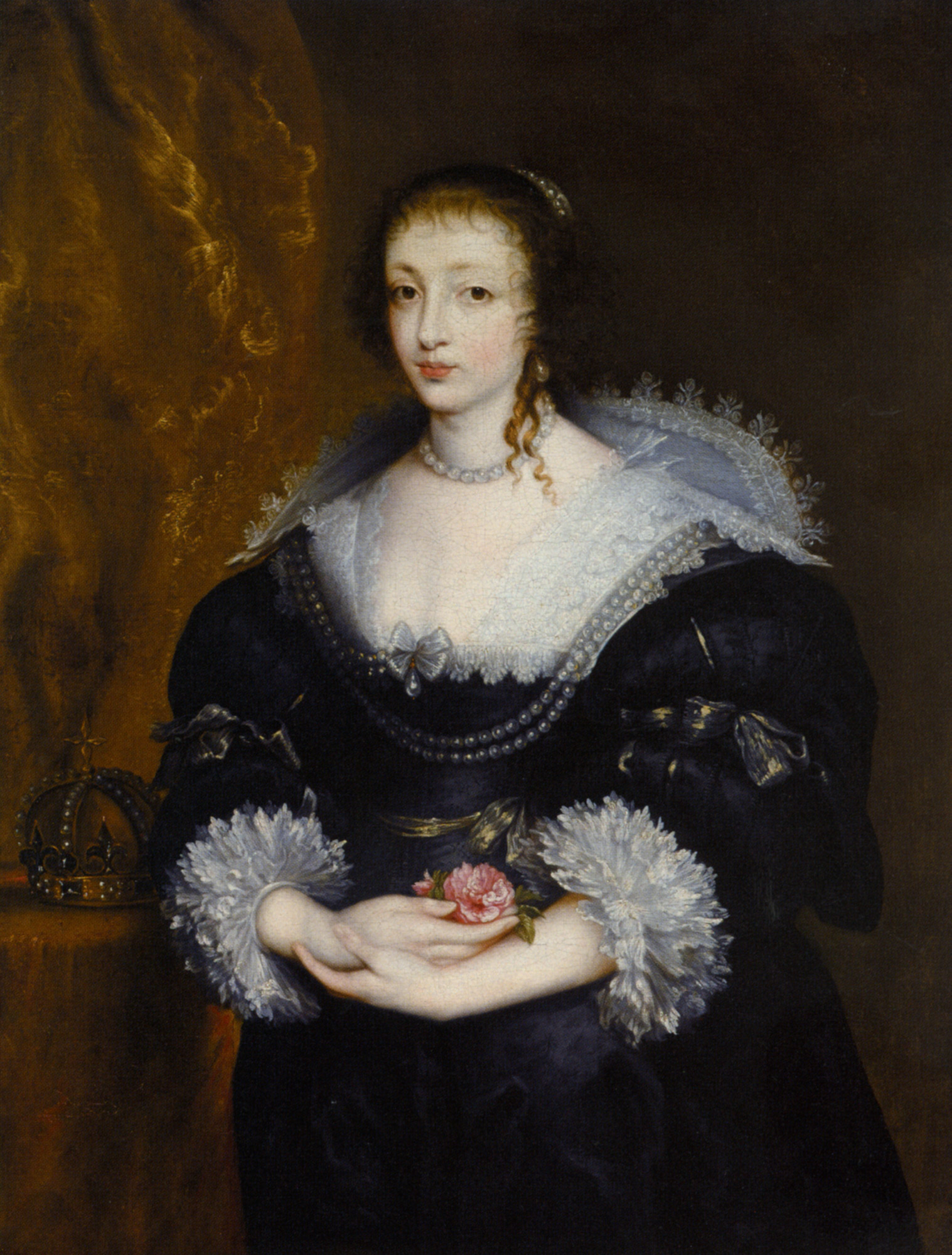This meticulously detailed portrait showcases a regal woman, possibly from the 16th or 17th century, depicted with exquisite realism. She stands elegantly, slightly facing to the left with her head turned slightly to the right, capturing a subtle, neutral expression. Her fair complexion and dark brown eyes are framed by her long, curly brown hair, which flows down to the top of her forehead, with a single sliver cascading down to her neck, obscuring her ears. 

Adorned in a voluminous, navy or black dress with intricate white lace trimmings on the shoulders and cuffs, the woman's attire is characterized by its heavy fabric and opulent design. A prominent bowtie graces the center of her chest, complemented by a strand of pearls draped over the dress. Around her neck lies an off-white pearl necklace. The ends of her sleeves feature puffy white fabric, adding to the dress's lavishness. Her hands are clasped gracefully at her waist, holding a red flower, likely a rose or carnation.

The background is a deep, rich brown, slightly lighter on the left side, where streaks resembling upward-facing lightning add dynamic texture. On the bottom left corner rests a table holding a black crown adorned with a gold star and numerous jewels, signifying her royal stature. This painting is a testament to the artistic skill of the era, with its remarkable attention to detail and the lifelike, soft rendering of the subject's features.